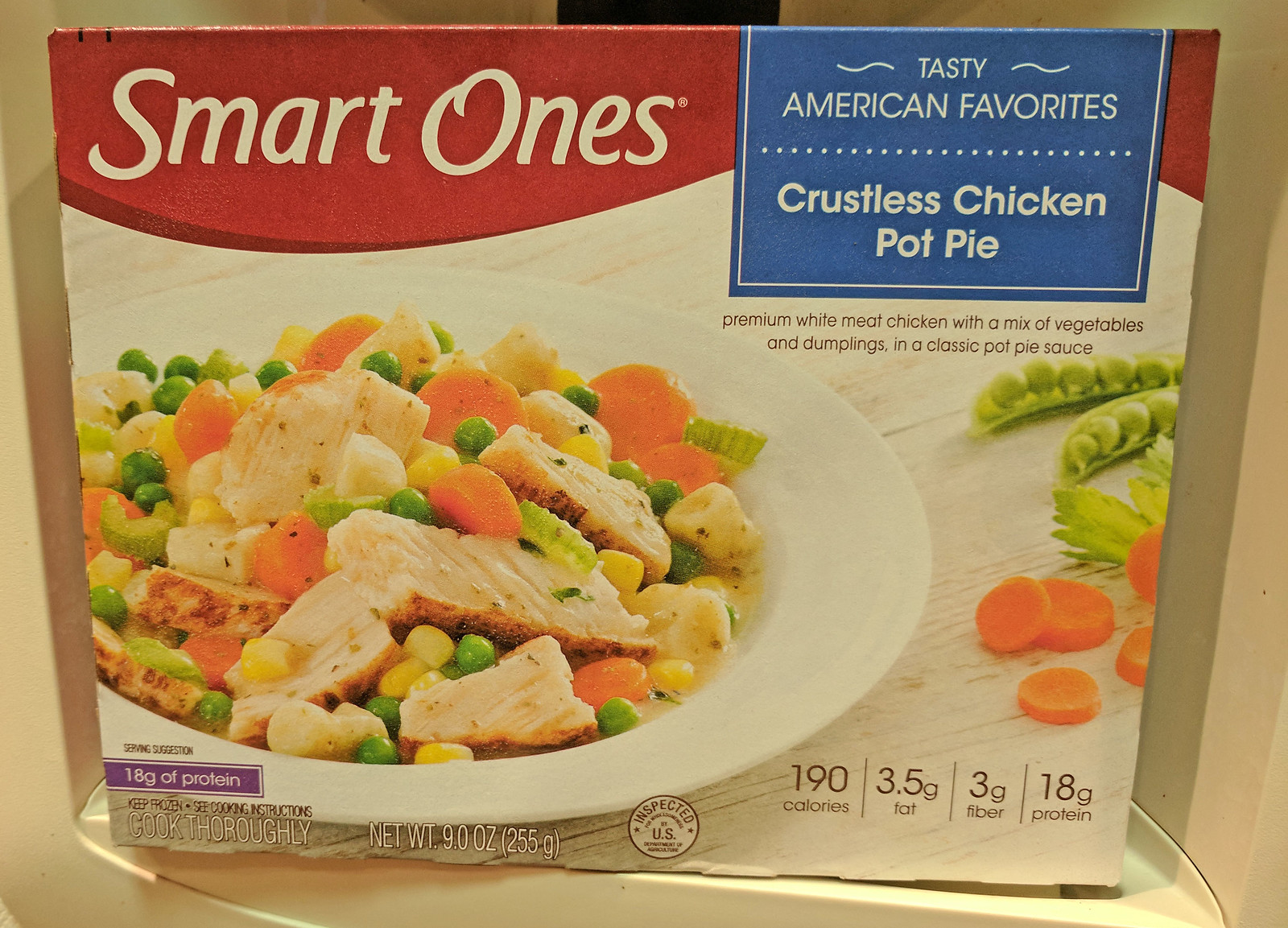The image portrays a box of a frozen meal, positioned upright to display its contents and branding clearly. The top of the box features a wavy red banner with white lettering that reads, "Smart Ones." In the upper right corner, there is a blue square with white text that states, "Tasty American Favorites." The featured dish is labeled as "Crustless Pot Pie."

Adjacent to this, you can see a spread of accompanying green peas and sliced carrots, accentuating the meal's ingredients. The main visual focus is on the dish itself, presented on a pristine white plate, showcasing sliced chicken, along with visible carrots and peas embedded in the pot pie.

In the bottom right corner of the box, nutritional information is clearly displayed: "190 calories," "3.5 grams of fat," "3 grams of fiber," and "18 grams of protein."